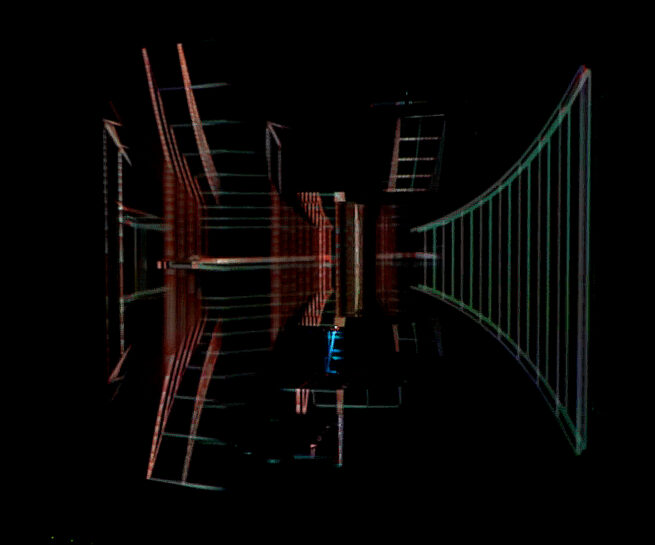The image appears to depict a complex graphic likely created on a computer, featuring a dynamic array of vividly colored lines set against a black background. Predominantly, these lines are green on the right side and red, with hints of blue, scattered throughout. The lines, seemingly in motion and diverging in various directions, give the impression of forming a large cylindrical room or tunnel-like structure. Adding to this, the image includes what seems to be a pedestal or screen positioned upfront, possibly serving as a control point for the light projection. The green sections form the edges of the cylindrical room, while red elements suggest a hallway-like passage, creating a mesmerizing, almost satellite-like appearance while resembling a light projection in an abstract, intricate setting.